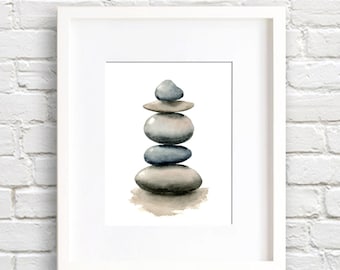The image features a small, horizontally oriented photograph of a framed illustration on a white brick wall. The thick white frame encloses a painting of five rocks, meticulously stacked upon one another. The painting is set against a generous light blue mat, enhancing the visual appeal. The rocks range in color from light brown to medium gray. At the base, the largest stone is flat and light brown. A smaller, medium gray stone sits atop it, followed by a larger, rounder, light brown rock. Above this, there is a flatter, light brown stone, and the stack is crowned with a small, gray rock. The illustration, which has a white background, also features a subtle light brown shadow beneath the rock stack, giving it a grounded appearance. The white brick wall behind the frame is clearly visible on either side, adding to the aesthetic with its textured surface.